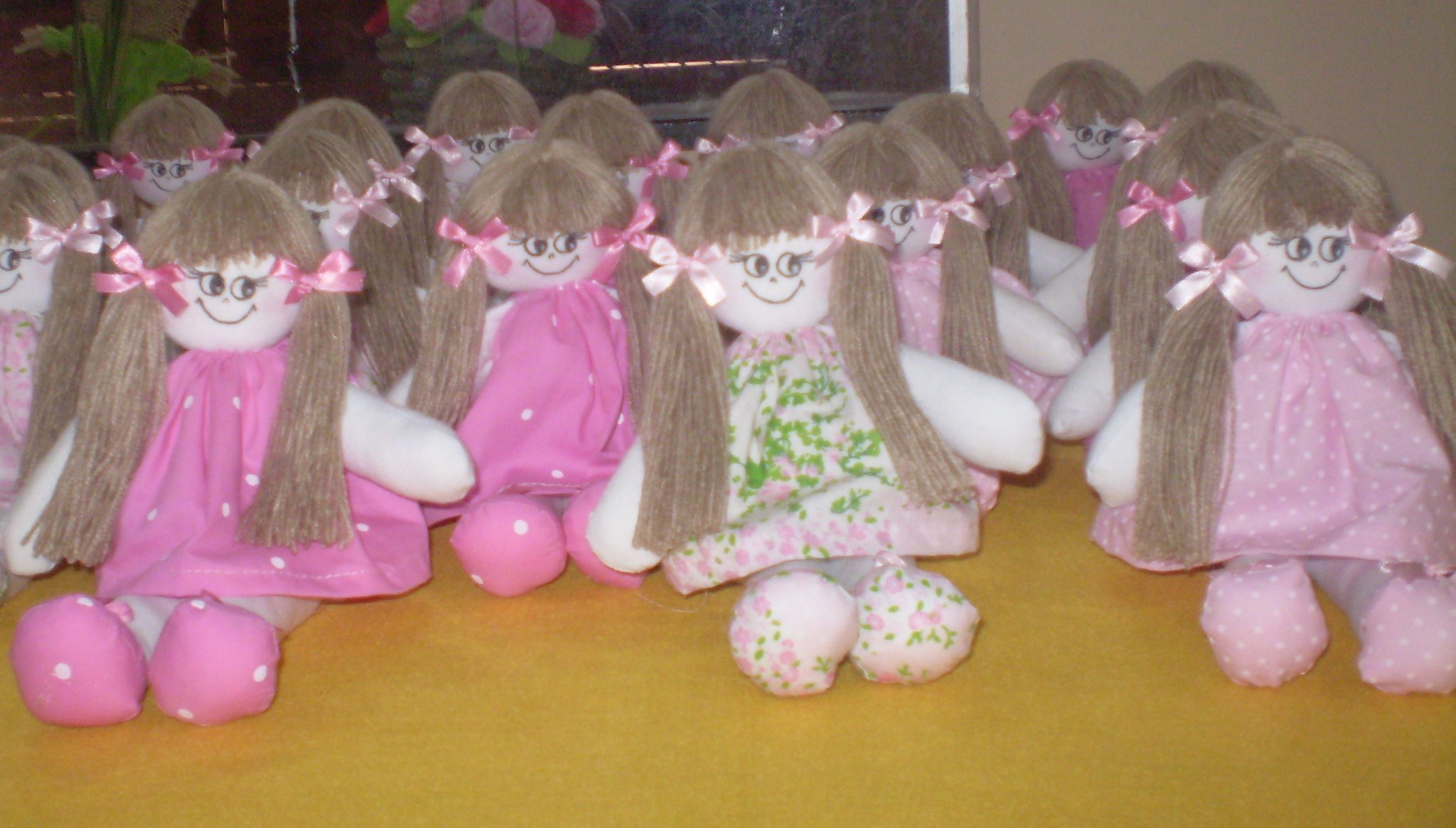This image showcases a complete collection of homemade dolls, arrayed on a light brown varnished table. Each doll features a similar face, characterized by painted smiles, dot noses, and eyes with prominent, diagonally-pointing eyelashes gazing off to the side. Their hair, made of high-quality yarn in shades of greenish-brown to golden-brown, is styled into large pigtails tied with pink ribbons and cut straight across the forehead.

The dolls' attire varies, yet maintains a cohesive theme. Their dresses range from bright pink with white polka dots to light pink with subtle white dots, and even whitish-pink with green floral designs resembling scattered leaves. Matching their dresses, their feet are similarly patterned, with pink and white polka dots or white featuring green sprigs reminiscent of parsley leaves.

In the background, a window adorned with drawings of plants adds a touch of charm to the scene. Each doll's rounded arms and legs enhance their endearing, homemade appeal, and their coordinated outfits and hairstyles evoke a nostalgic connection, recalling designs familiar from childhood collections.